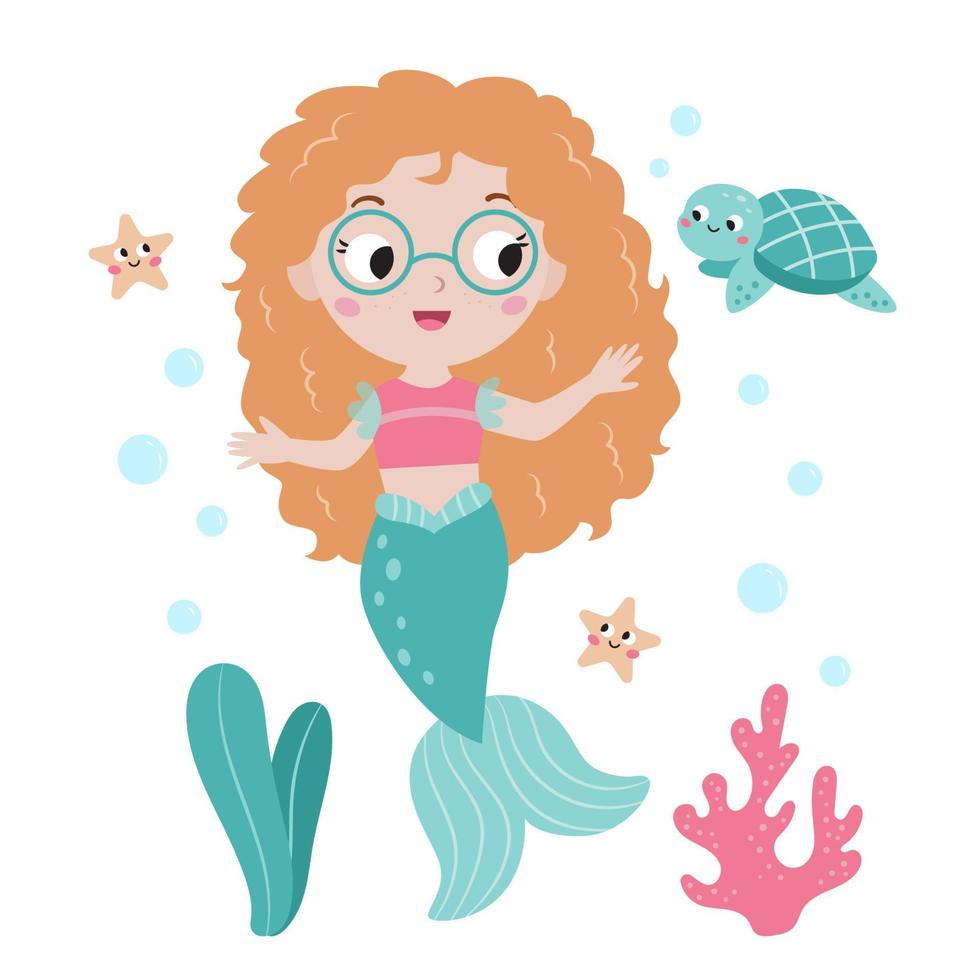This is a detailed cartoon image of a cheerful young mermaid facing forward with outstretched arms, giving the impression that she is floating joyfully in the water. She has long, curly brown hair and wears teal round glasses. Her expressive eyes feature large white sclera with black pupils looking to her left (our right). She also has darker brown curved eyebrows, long eyelashes, an open smile revealing her teeth, and rosy cheeks marked by two small circles.

Her attire includes a pink crop top with semi-transparent teal ruffles around the shoulders, exposing her arms and belly area. Her mermaid tail is a striking turquoise with lighter turquoise at the end and accentuated with white curved stripes.

Surrounding the mermaid are various sea elements, enhancing the underwater fairy-tale atmosphere: a smiling turquoise sea turtle to the upper right, a happy light brown starfish to the upper left, two green leaves in the lower left corner, and pinkish-red coral dotted with little dots in the lower right corner. Additionally, there are small bubbles scattered around her, adding a whimsical touch to the scene.